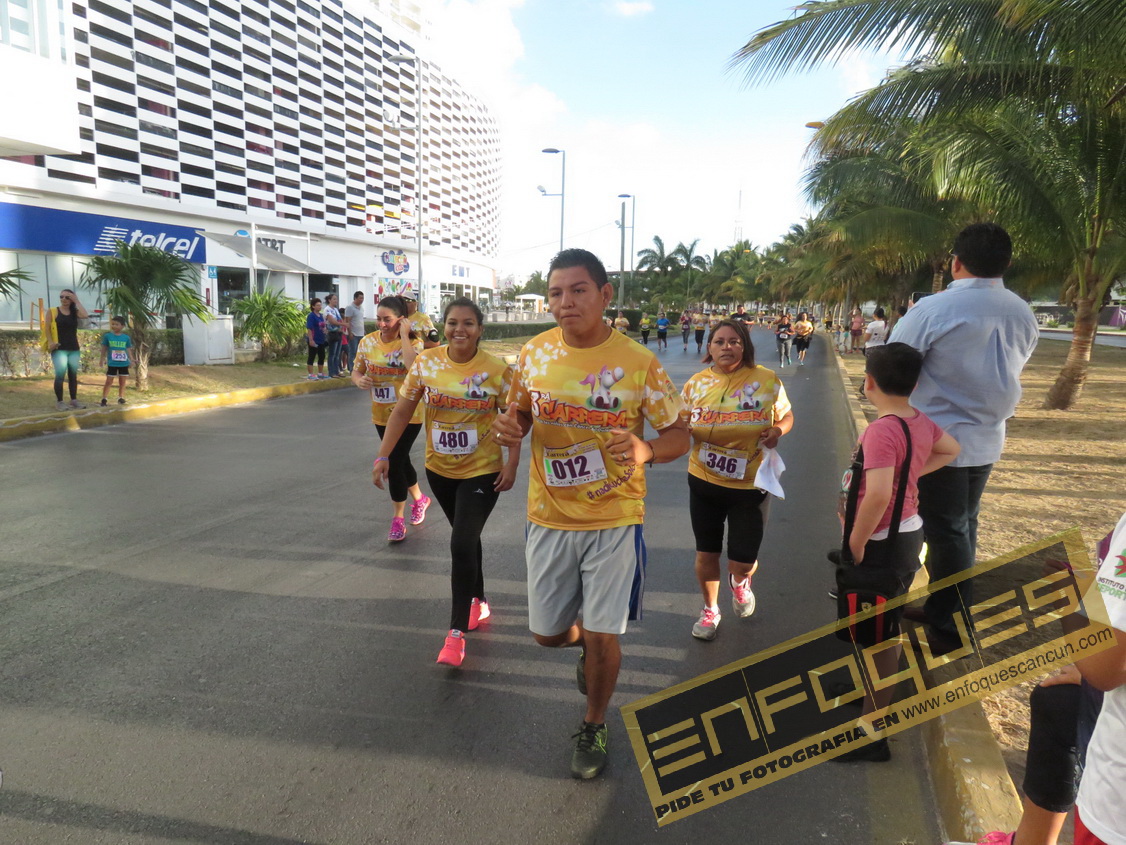The image depicts a vibrant outdoor scene of a marathon or charity walk. In the foreground, four runners, all clad in yellow T-shirts with black numbers, are prominent. The group is running along a paved road, exuding a spirited and joyful energy. Among them, a young boy in a pink T-shirt and black shorts with a bag slung over his shoulder stands out. The left side of the image showcases a large white building with prominent "TELCEL" and "AT&T" logos, clearly situating the scene in Mexico. Also visible are rows of green palm trees that line the area, enhancing the tropical ambiance. Spectators can be seen to the right, standing and cheering from the sidewalk, underscoring the supportive atmosphere of the event. To the bottom right, the watermark "ENFOQUES PIDE 2 PHOTOGRAPHYEN WWW.ENFOQUESCANCUN.COM" authenticates the photo, hinting at its professional capture. The blue sky overhead, the well-lit road, and additional details like lampposts and dirt pathways combine to create a vivid and dynamic snapshot of the lively event.